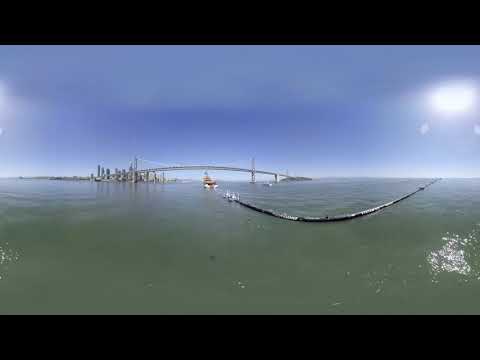The photo captures a vibrant scene taken out at sea with milky green water extending across the bottom half of the image. A bright white sun hangs in a cloudless, clear blue sky, casting its light over the expanse. Dominating the center of the image is an orange boat seemingly pulling a curved rope that runs from the bottom right across the scene. In the distance, a large arched driving bridge gracefully stretches from the left to the right side of the image. To the left of this bridge, towering skyscrapers and tall buildings define a bustling city skyline, possibly reminiscent of Miami or a similar coastal city. Nearby, an additional small boat is seen navigating towards the bridge. The right side features a smaller island, completing the picturesque maritime vista.